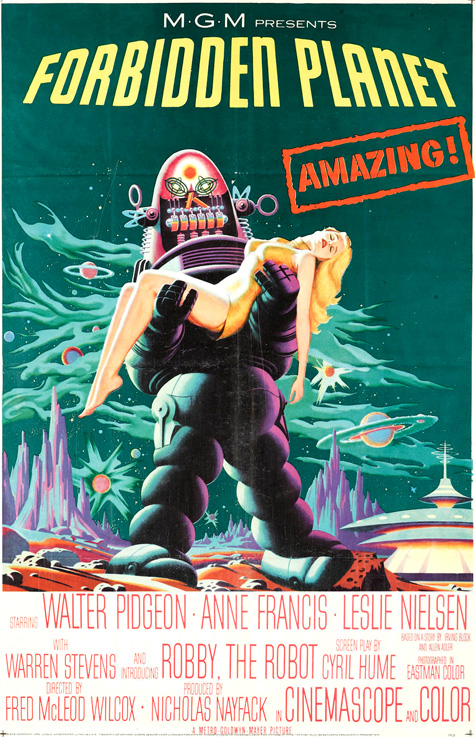This is a detailed movie poster for "MGM Presents Forbidden Planet." Dominating the top center in bold yellow letters are the words "Forbidden Planet," with "MGM Presents" just above it. To the right, "Amazing" is displayed in striking red letters within a rectangular red border. The primarily blue-green background sets a space-like setting featuring green wispy clouds, planets with rings, blue mountains or towers, and a red, alien surface. The focal point is a prominent purple robot, reminiscent of the one from "Lost in Space," carrying a blonde, white woman in a small gold dress, who seems either unconscious or asleep. A futuristic building is also visible in the background. The lower half of the poster lists cast and credits in red letters against a white background: Starring Walter Pidgeon, Anne Francis, and Leslie Nielsen, with Warren Stevens and introducing Robbie the Robot. Additional credits note Cyril Hume for the screenplay, Fred McLeod Wilcox as the director, Nicholas Nafak as the producer, and it highlights the film being presented in CinemaScope and Eastman Color.